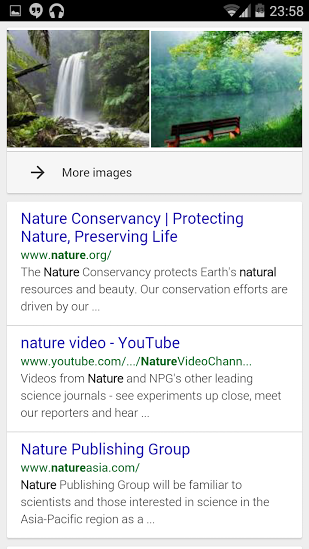Screenshot of a Mobile Phone Display:
 
At the top, a black status bar contains several icons including a camera, conversation bubble, share symbol, network signal, battery indicator, and the time "23:58."

Below the status bar, two images are prominently displayed. The first image depicts a majestic waterfall cascading through a lush, verdant rainforest. The second image features a tranquil rainforest scene with a solitary park bench nestled among dense foliage.

Directly beneath these images is a white banner with the text "More images" accompanied by a right-pointing arrow, suggesting additional images can be viewed.

Further down, there are three listings:

1. **Nature Conservancy: Protecting Nature Preserving Life** 
   - **Website**: [www.nature.org](http://www.nature.org) (the URL is highlighted in green).
   - **Description**: "The Nature Conservancy protects the Earth's natural resources and beauty. Our conservation efforts are driven by our..."
   
2. **Nature Video - YouTube**
   - **Website**: [www.youtube.com/naturevideochannel](http://www.youtube.com/naturevideochannel) (the URL is highlighted in green).
   - **Description**: "Videos from nature and NPGs from other leading science journals. See experiments up close. Meet our reporters and hear..."
   
3. **Nature Publishing Group**
   - **Website**: [www.natureasia.com](http://www.natureasia.com) (the URL is highlighted in green).
   - **Description**: "Nature Publishing Group will be familiar to scientists and those interested in science in the Asia Pacific region as a..."

Each listing is characterized by blue titles and green URLs, with descriptive text providing a brief overview of their mission and content.